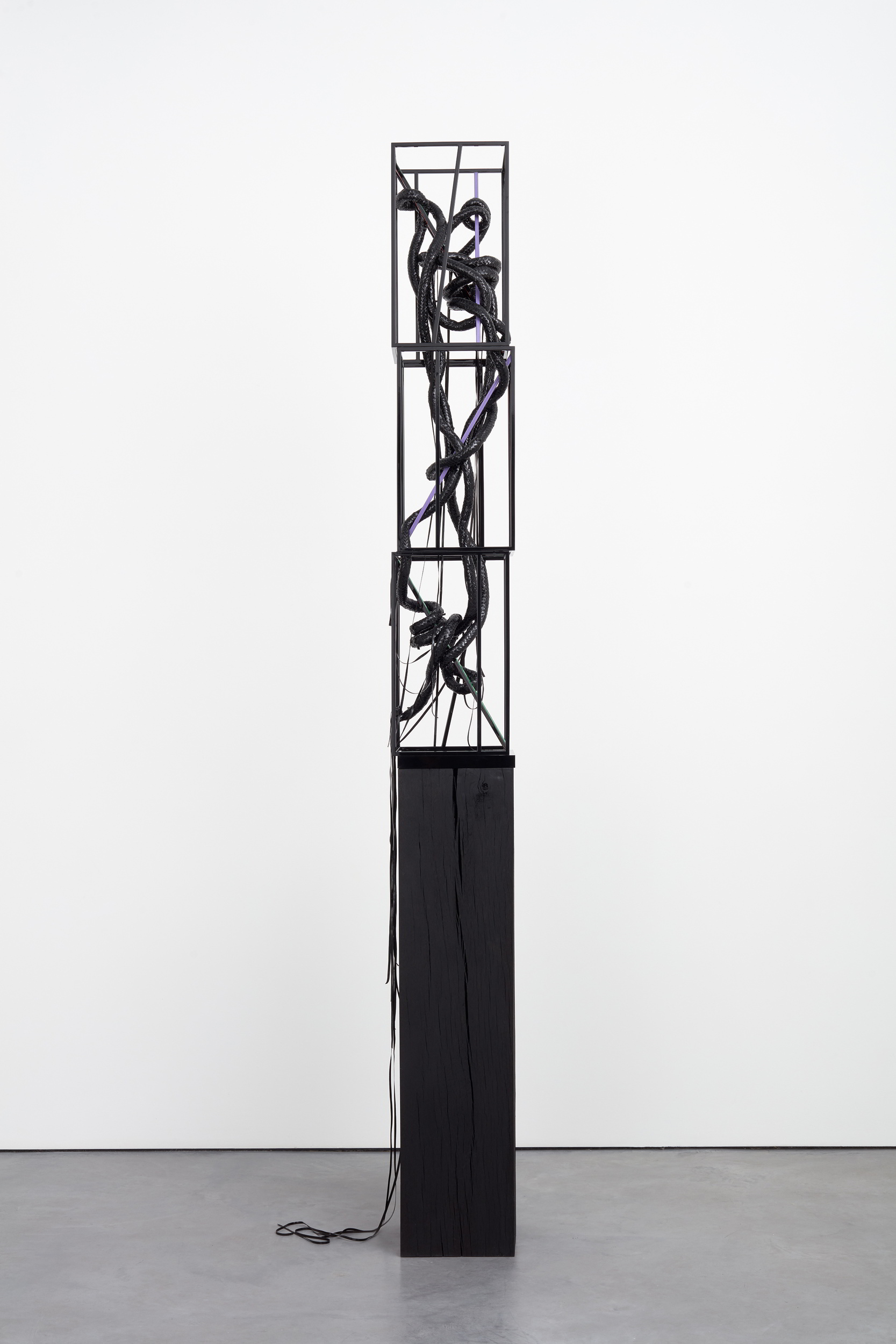This is a black-and-white photograph of an abstract art piece displayed in a museum. The piece features a solid, dark rectangular base a few feet high, set against a light-colored floor and a white wall. Rising from this base are three rectangular metal structures, stacked slightly askew atop one another, creating a tall, slender framework several feet higher than the base. Interwoven within these metal rectangles is a tangled, twisting mass of dark materials, possibly resembling rope or vine, that appears to be melting or withering. Some elements of this tangled structure dangle down to the floor. The top portion of the artwork includes transparent sections, allowing a view through to the white wall behind it, enhancing the intricate and somewhat pretentious appearance of the piece.